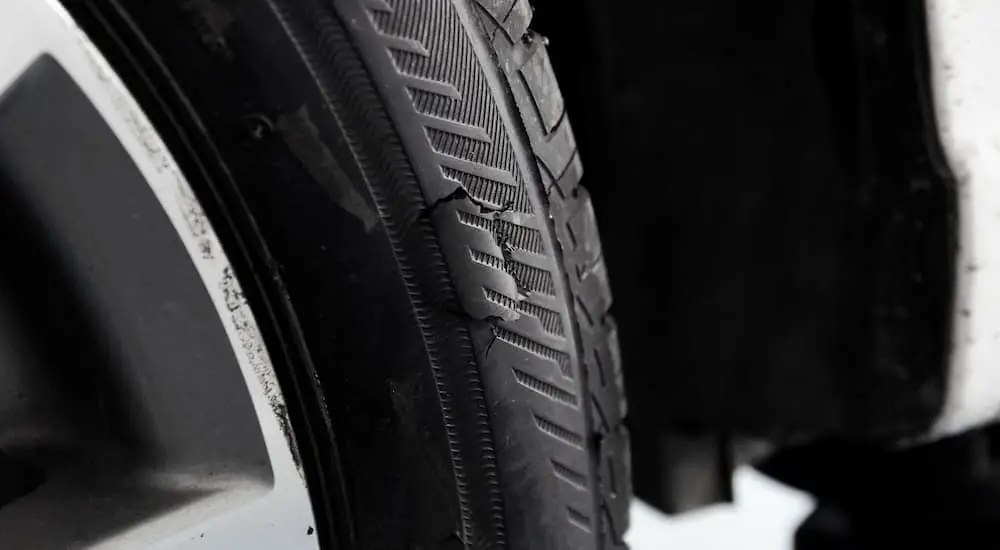The close-up, black-and-white photograph features a detailed image of a damaged car tire. The tire itself, which is black with a relatively new tread, has a noticeable rip or chunk missing from its surface, situated prominently in the center of the frame. Although the tire appears fairly new and is not worn out, the damage is severe and clearly visible. Part of the silver-colored rim is visible on the left side, showing minimal signs of wear. In the background, parts of the car are slightly visible, including what seems to be the metal bumper or frame of a white or gray vehicle. The lighting accentuates the tire's texture and damage, contrasting against the muted, grayscale backdrop.